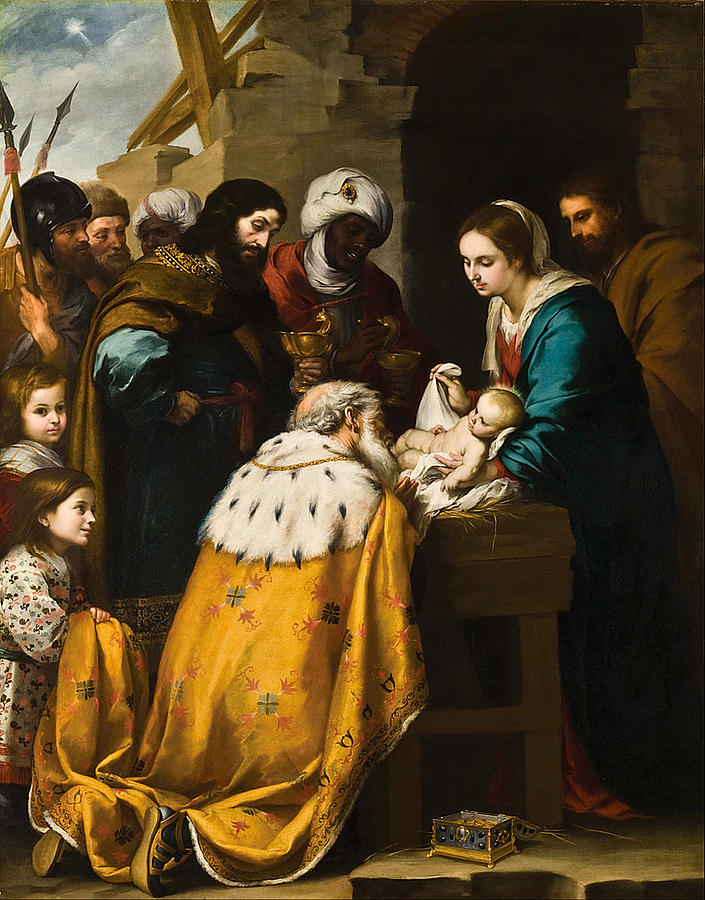This detailed portrait oil painting, titled "Adoration of the Magi," by Bartolome Esteban Murillo, originates from the 17th century and exemplifies the Baroque style. The scene portrays the biblical nativity with the Virgin Mary, dressed in a blue gown with a white cloth on her head, standing on the right. Behind her, Joseph wears a yellow shroud. Mary holds the naked Christ child, swaddled in a white cloth, in her arms, revealing him to an adoring wise man who is kneeling before them. This wise man is distinguished by his long gold robe adorned with an ermine fur collar, gray beard, and bald top. 

Another wise man with dark hair and beard, draped in a brown robe and blue undershirt, stands behind, alongside a dark-skinned man in a white turban and scarf with a burgundy robe. Both admire the baby Jesus, possibly holding chalices as if in offering. Behind this central group are several onlookers who contribute to the scene’s depth. Two small children are seen gazing at the child from the bottom left corner, while a small chest of jewels lies on the ground at the bottom right, hinting at the gifts of gold, frankincense, and myrrh. 

The background reveals a rustic barn made of stone and wood, indicative of the stable setting of Jesus's birth. Above, a sparkling star illuminates the sky, symbolizing the Star of Bethlehem that guided the wise men. The painting's artistic finesse and rich narrative reflect Murillo's masterful depiction of this profound religious moment.